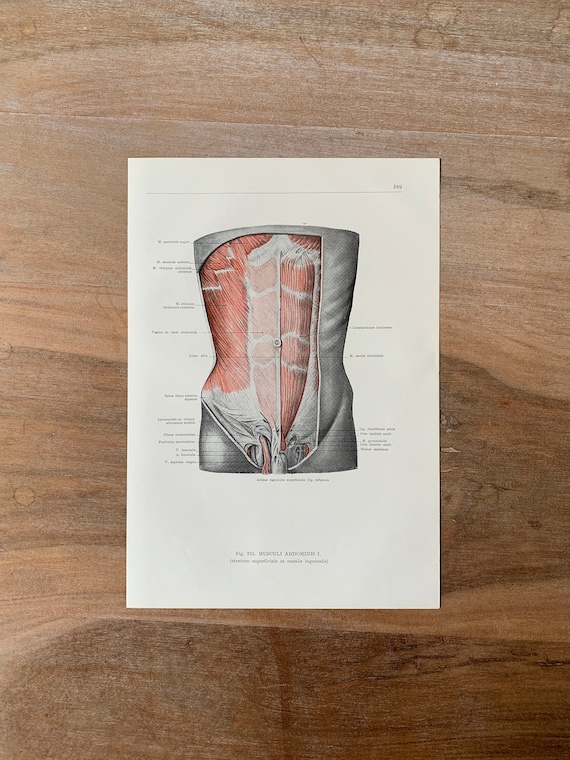The image is a vertically oriented, realistic photograph depicting either a wooden wall or floor as the background, creating an ambiguous perspective. Placed against this wooden backdrop is a large beige-colored page, seemingly torn from a medical textbook and identified by the number 149 in the top right corner. This page features a detailed anatomical diagram of a human torso, focusing specifically on the area from the top of the ribs down to the groin. The diagram appears to be hand-drawn, although possibly enhanced with computer animation, and portrays an intricate view of the abdominal muscles. The muscles highlighted in the illustration are rendered in pinkish-red, while the rest of the torso is shown in gray to represent the skin. Black lines and text attempt to label various anatomical elements, although the font is too small and blurry to be legible. The lower part of the page bears the text "muscle abdominis," reinforcing the focus on abdominal anatomy. This descriptive medical diagram serves to illustrate the muscle groups and inner workings of the human torso, making it a likely feature in a technical fitness manual or anatomy book.